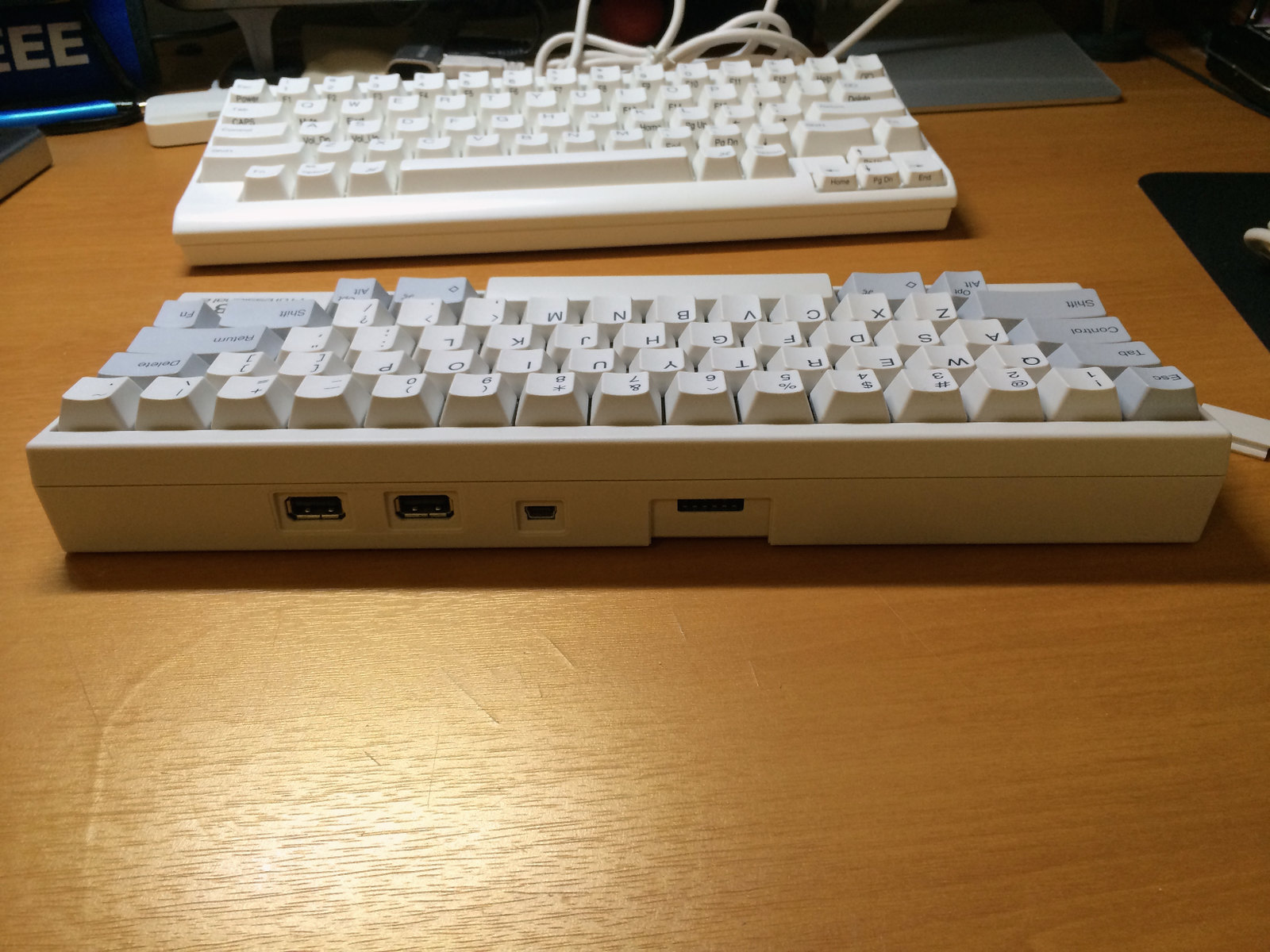This color photograph, taken from a top-down perspective in landscape format, showcases two computer keyboards placed on a light brown, somewhat scratched-up wooden table. Both keyboards are predominantly white, though the one positioned at the bottom of the image has larger, clunkier keys, indicative of an older model, and some of its keys are gray. The keyboard at the top of the image also features some gray keys and numerous tangled white cables extending from it. The keyboards are oriented towards each other, with their spacebars facing inward. A blue pen is positioned near the top keyboard, seemingly pointing at it. There are various other items on the table, including what appears to be a black and gray mouse mat to the upper right and a dark object with "EE" written in white capitals and a line of bright blue, possibly neon, illumination. The photograph also reveals, above the top keyboard, four connectivity ports on the back, adding to the detailed and cluttered scene.